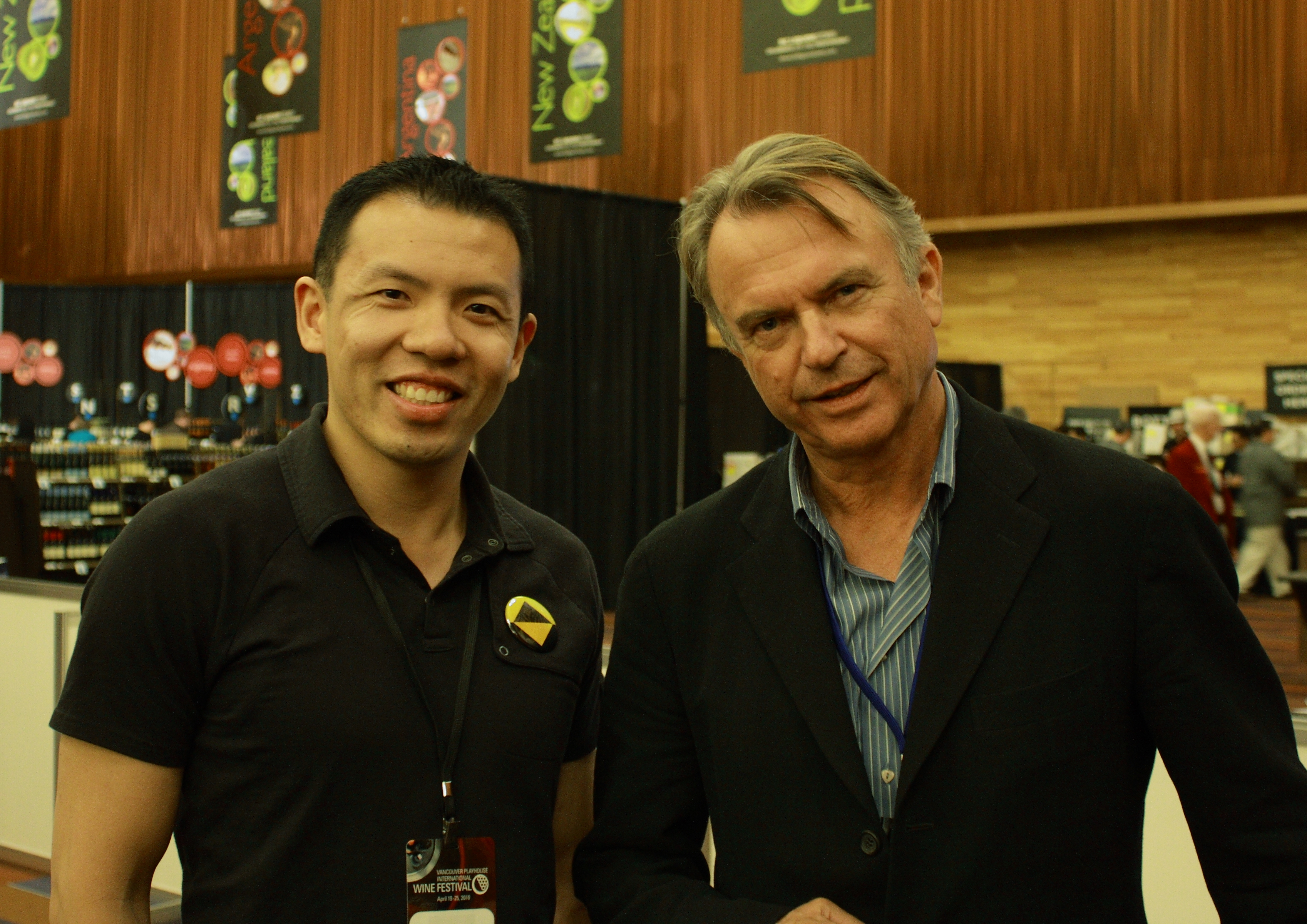This color photograph features two men, one of whom is the actor Sam Neill, famous for his role in Jurassic Park, standing side by side at what appears to be a convention or festival event. On the left is a young adult Asian male with short black hair, beaming broadly. He is dressed in a black polo shirt with a small yellow and black symbol on the left chest and wears a black lanyard around his neck, clipped to an identification badge that reads something about a wine festival. To his right stands Sam Neill, with medium-length brown hair, slightly cocking his head to the left and wearing a reserved smile. Neill is dressed in a black blazer over a blue button-down shirt and a blue lanyard that is partially hidden under his jacket. Both men are looking directly into the camera. The background reveals a busy setting with various booths, a brown wall adorned with posters and banners, a wood floor, and a few people walking by, further suggesting a lively convention atmosphere.